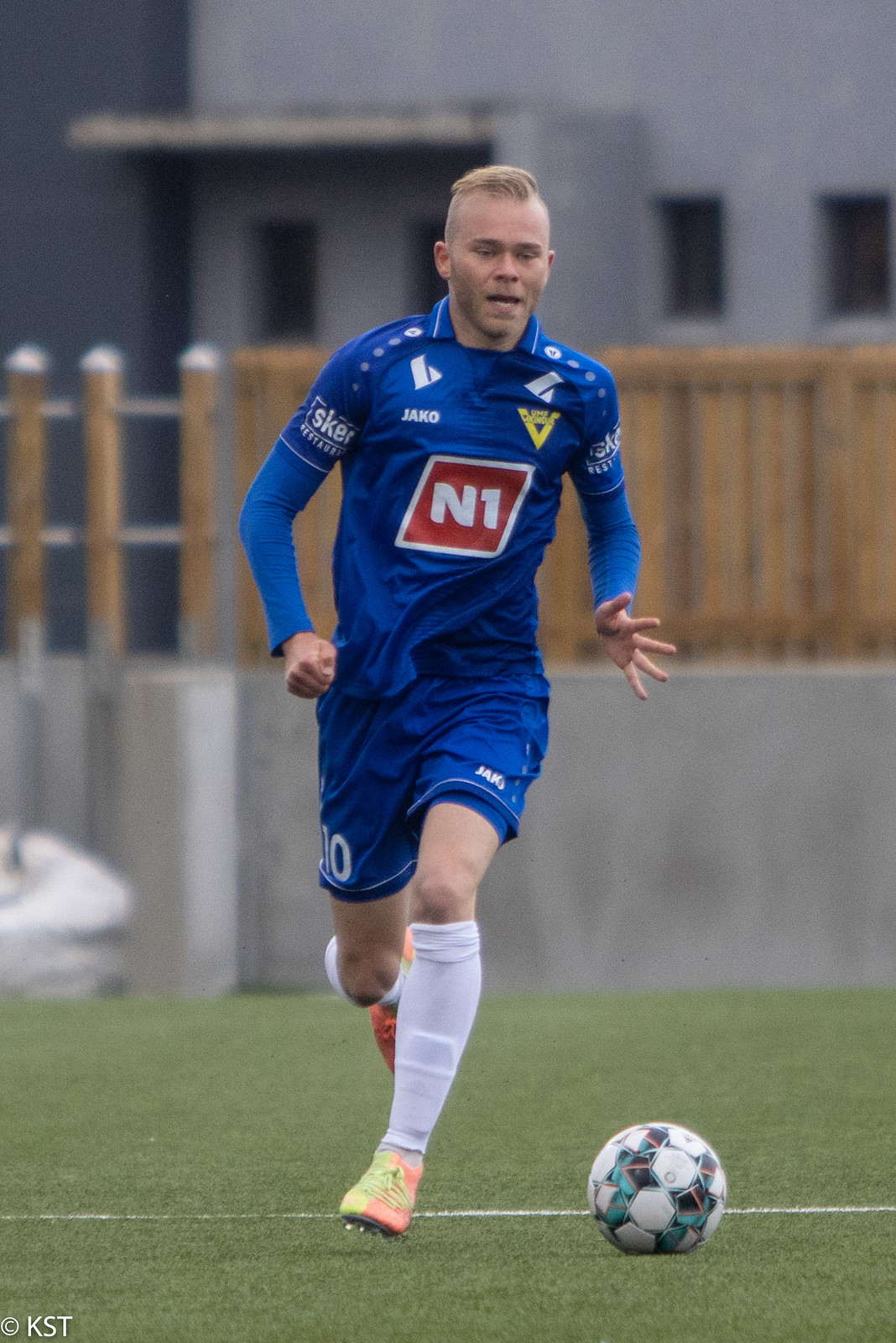This photograph captures an action-packed moment on a sports field set outdoors, most likely in the middle of the day. At the center of the image is a man running towards the camera, dressed in full football gear. He has short blonde hair, shaved on the sides and slightly longer on top. He sports a blue ensemble consisting of blue shorts, a blue collared jersey with a long sleeve shirt underneath, and white socks, one of which reveals a shin guard. His jersey features a prominent red diamond with the inscription "N1" in white lettering. His cleats are a striking combination of yellow and orange.

The lush green field, marked with painted lines, suggests a football or soccer field. A white, black, and green football is on the ground near him. In the blurred background, a stone wall with a wooden fence and a stone building can be seen, lending a sense of depth and context to the scene. The image includes a visible watermark with the initials "KST." The vibrant colors—white, green, yellow, hot pink, light blue, black, dark blue, red, brown—add to the dynamic feel of the photo.